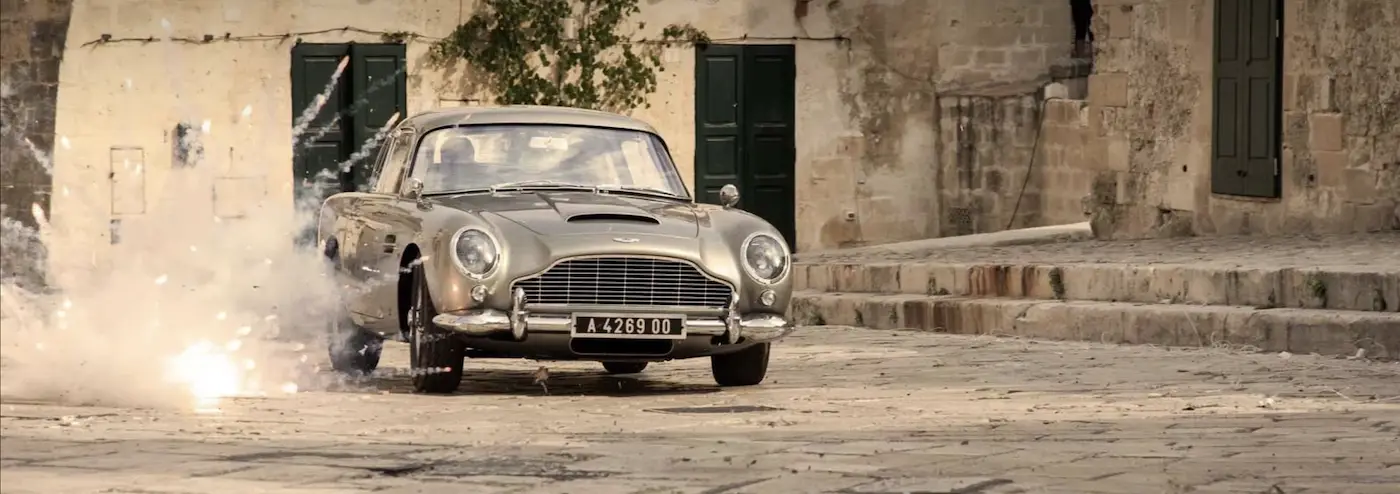In this action-packed scene, we witness an iconic silver Aston Martin DB5, famously associated with James Bond films, prominently centered and slightly to the left in the image. The car, with its chrome grille, bumper, headlight bezels, side mirrors, and rims, gleams as it speeds through what appears to be an old, abandoned place with cobblestone streets. The license plate reads A426900. To the left of the car, an explosion has just occurred, sending smoke and pebbles flying. On the right side, a set of stairs ascends between the old stone buildings. In the background, a brick wall flanked by black-painted doors and climbing vines is visible, with a solitary tree above it. The grayscale tones of the car, combined with the tan cobblestones, the muted green of the tree, and the surrounding stone structures, create a dramatic and thrilling atmosphere reminiscent of a high-stakes movie poster set in a historic European locale.